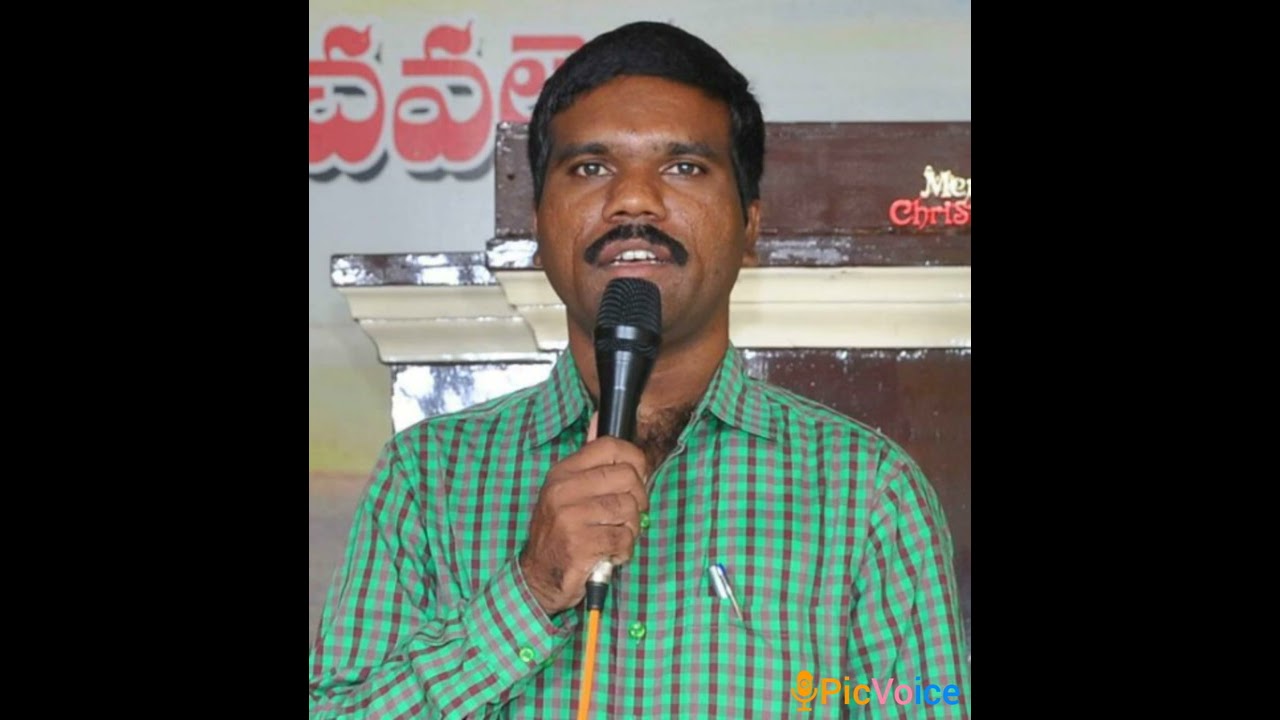The image depicts an Indian man with dark brown skin, short black hair, and a well-groomed mustache, speaking into a black microphone with a yellow cord. He has a wide nose and light eyes. The man is dressed in a long-sleeve, button-down shirt with a green and purple plaid pattern, accented by stripes of purple and brown. Notably, he has a pen tucked into the front pocket of his buttoned-up shirt, which reveals a hint of chest hair despite being mostly buttoned except for the top button. Behind him, an awning extends from a wall, and above that, some drywall is visible featuring Hindi text. There is also a neon sign in the top right-hand corner. In the bottom right of the image, there is a small webcam logo with the text "PIC" in yellow, "VO" in pink, and "ICE" in blue. The background includes what seems to be the top part of a fireplace mantel, possibly with a partially visible "Merry Christmas" sign.